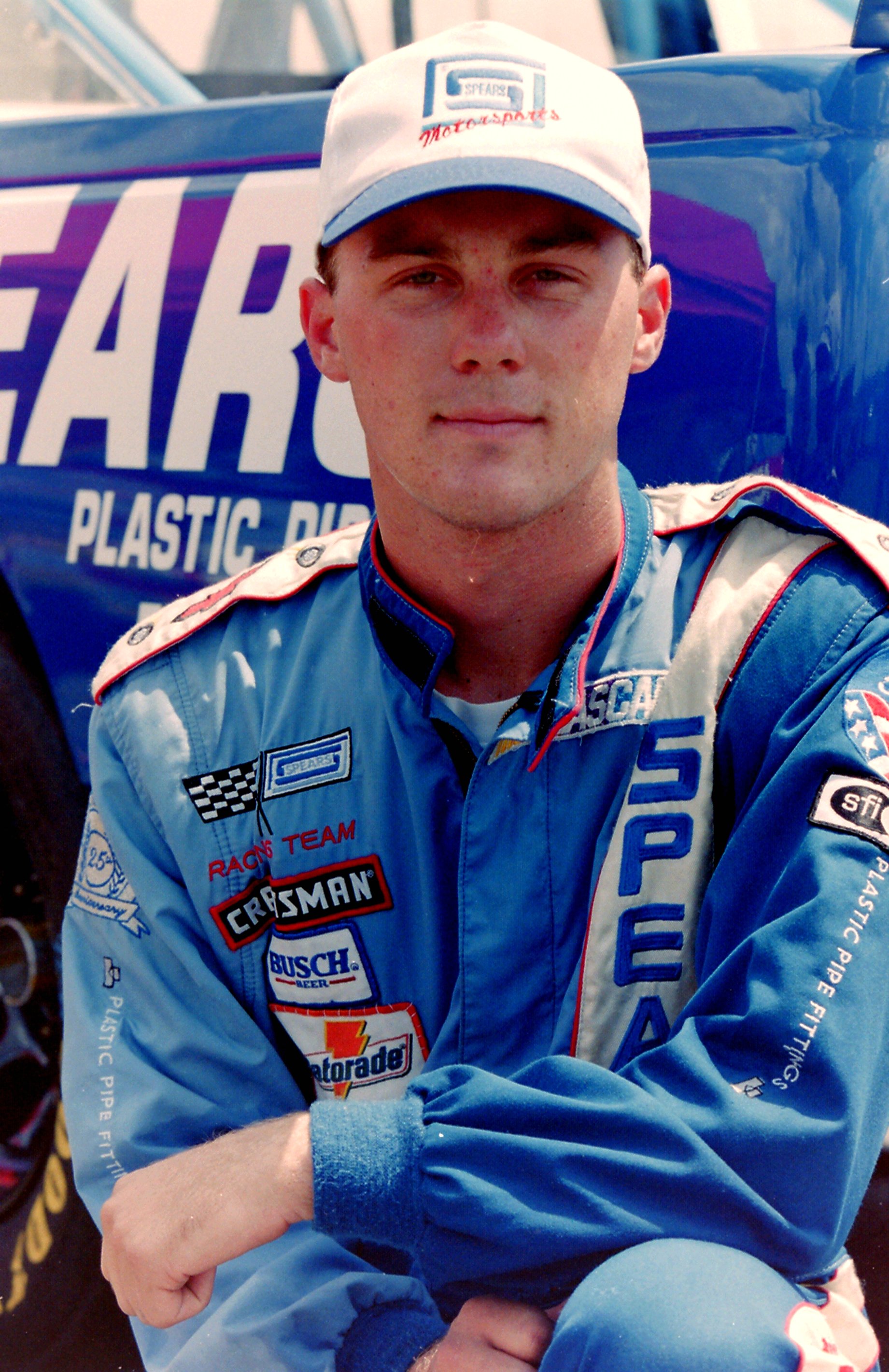In the image, a young Caucasian man, appearing to be in his early 20s, is squatting on one knee with his left arm resting on his left knee. He is dressed in a blue racing jacket adorned with various advertisements, including brands like Gatorade, Bush Beer, and Craftsman. The jacket also features a NASCAR label and a checkered flag emblem with the words "Race Team" beneath it. He is wearing a white and blue baseball cap with a logo and red writing, though the specifics are unclear. The man has short hair hidden under his hat, dark eyes, and bushy brown eyebrows. He is positioned in front of a blue vehicle, which likely correlates with his racing attire. The vehicle has partial visible text on it, reading "E," "AR," and "plastic," although the full context is obscured. The man is staring directly into the camera, exuding an air of confidence and professionalism.